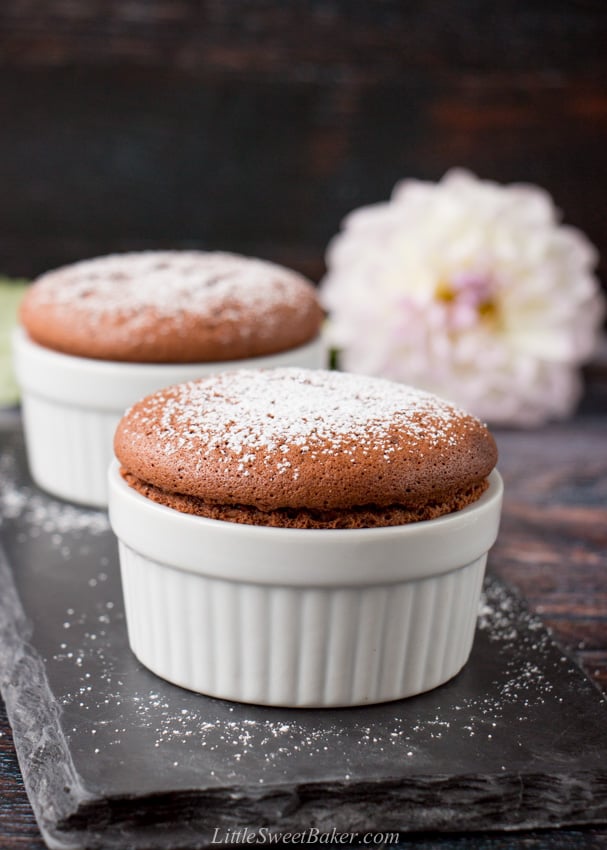This photograph, sourced from littlesweetbaker.com as indicated by the watermark at the bottom, captures an enticing scene of desserts. The image, in portrait orientation, features two white ceramic ramekins, each containing a chocolate brown cake. The cakes, likely souffles or muffins, rise about an inch above the ramekin rims and boast a dusting of powdered sugar, some of which has landed gracefully on the surrounding dark slate or black marble surface. The foreground ramekin is centered, with the second ramekin positioned diagonally behind and to the left. In the upper right corner, a blurred white flower, possibly a peony or dahlia, adds a delicate touch to the composition. The backdrop includes a blurred, grainy texture with hints of dark black and occasional brown, enhancing the warm and inviting atmosphere of this dessert display.